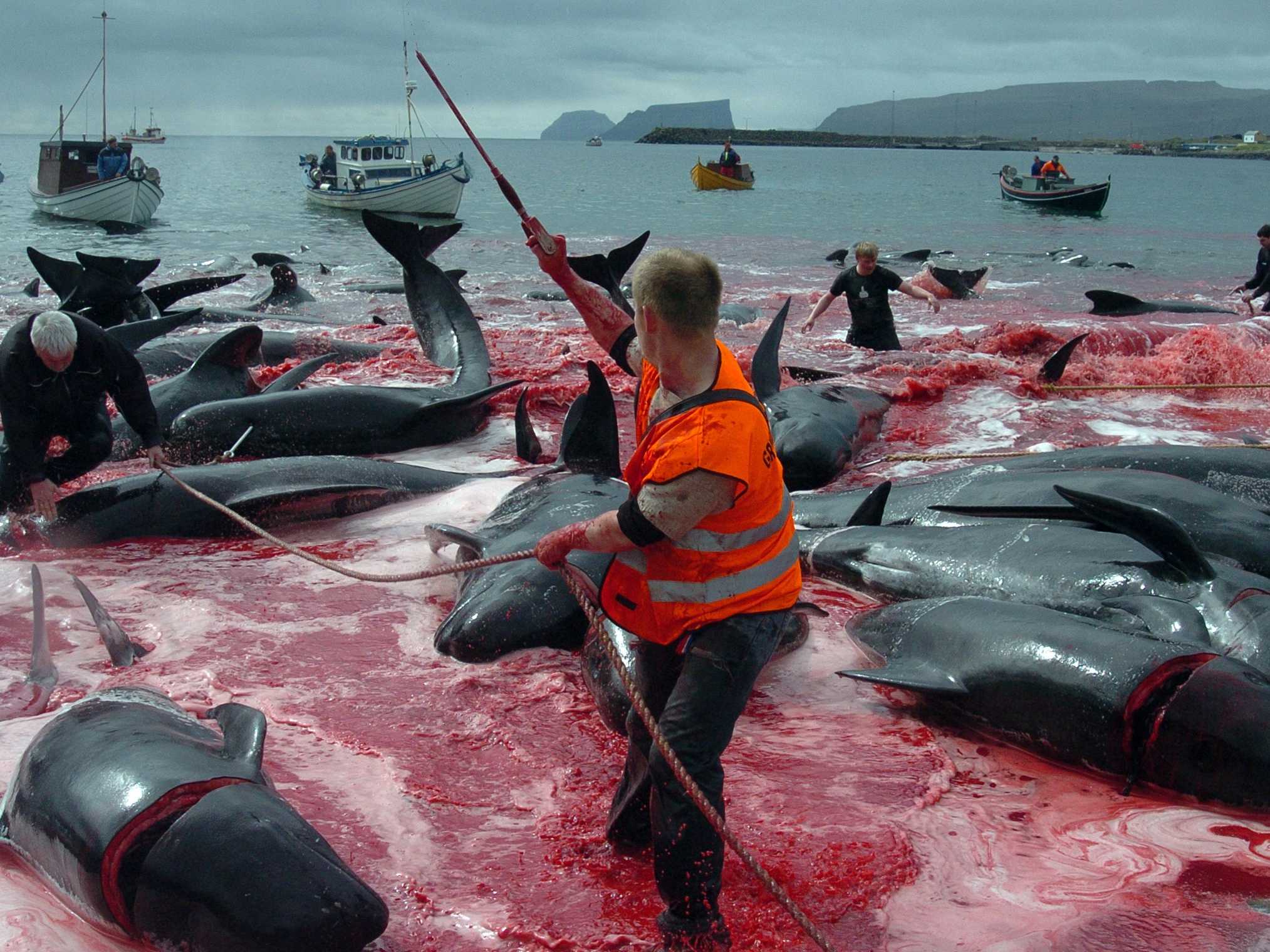On a shoreline, a group of fishermen is engaged in the gruesome task of slaughtering and processing multiple black whales, each roughly the size of dolphins. The whales, identifiable by their rounded noses, lie in various stages of being butchered, with many of them still impaled by harpoons and their heads partially severed. The scene is saturated with blood, with the water near the shore turned red. In the foreground, a man, wearing black pants, an orange safety vest over a tan short-sleeved shirt, and covered in blood, is visible from his ankles upwards as he pulls on a thick rope attached to a harpoon embedded in a whale further away. The harrowing backdrop includes fishing boats and additional fishermen, all contributing to the starkly brutal tableau of the blood-splattered ocean scene. The air is thick with a sense of grim determination as these fishermen work within a starkly industrial yet disturbingly violent atmosphere.